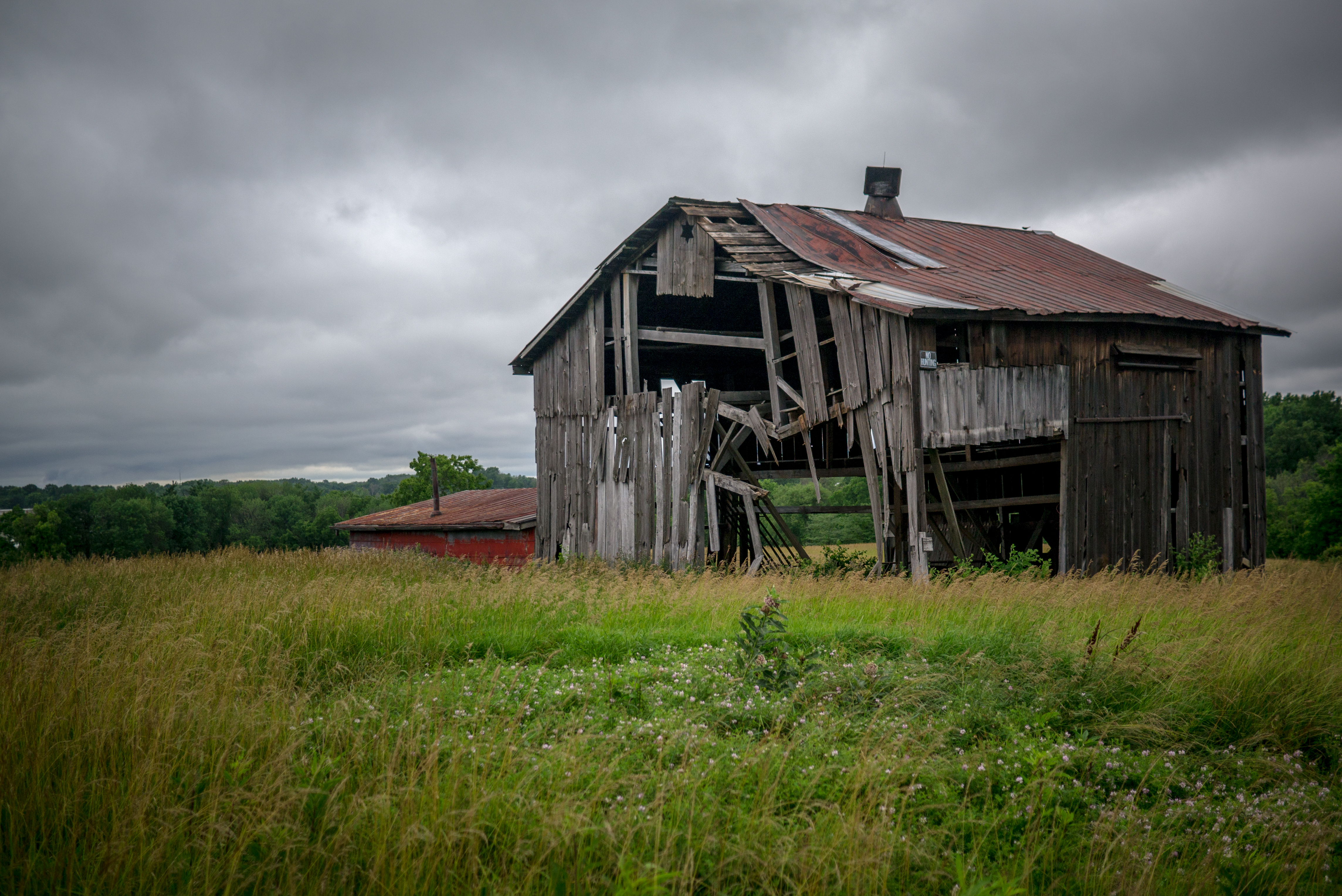A captivating photograph features an old, dilapidated farmhouse, constructed with weathered wooden planks now visibly rotten and broken. The house is topped with a rusty, zinc metal roof, crowned by a prominent, protruding chimney. The structure stands amid an overgrown, grassy farm, where patches of wildflowers add a splash of color to the otherwise green landscape. To one side of this abandoned relic, a newly built, reddish house also featuring a chimney contrasts starkly with its worn surroundings. The background is filled with large, verdant trees, their greenery a testament to the vitality juxtaposed against the house's decay. Overhead, the sky is laden with dark, grey clouds, hinting at an impending storm or the onset of winter, creating a moody and atmospheric scene.